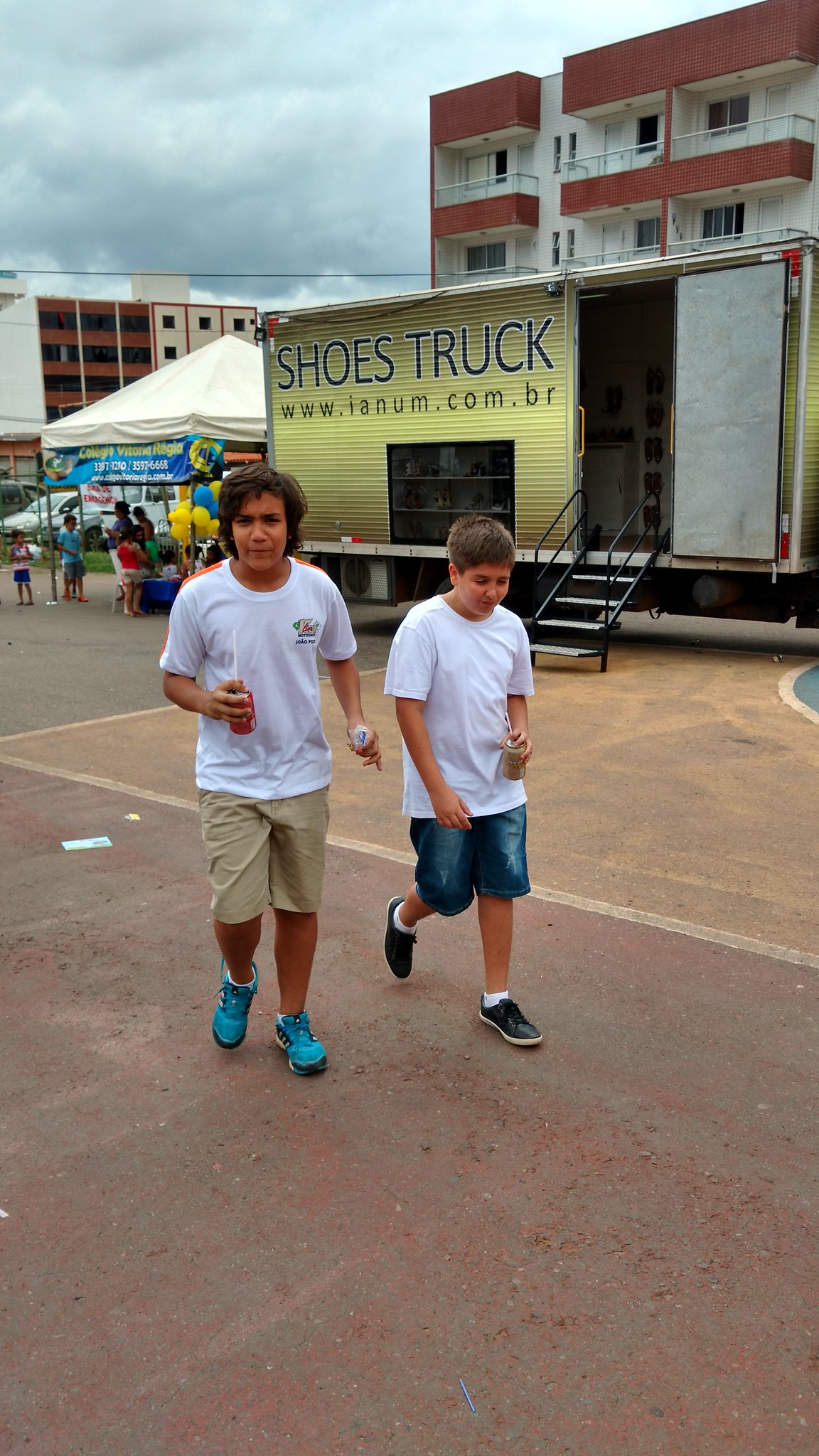The image captures two young boys, one slightly taller than the other, who appear to be of Latino or possibly white descent. They are walking side by side down a street or possibly at an outdoor festival. The taller boy on the left has brown hair and is wearing a white t-shirt, khaki-colored shorts, and blue tennis shoes. He holds a soda can in one hand and another object in the other. His companion on the right, who could be either Latino or white, is similarly dressed in a white t-shirt, denim shorts, white socks, and black shoes. This boy carries a cup with a straw as they stroll along.

In the background, a green trailer marked "Shoes Truck" and the website "www.inem.com.br" is visible, with a ladder extending from its side and an open door. Adjacent to the trailer stands a booth adorned with blue, yellow, and white balloons, topped with a matching banner. This booth seems to attract a crowd of both children and adults. Behind the bustling scene, high-rise apartment buildings of white and brown hues reach into a cloudy sky, suggesting an overcast day with no visible sun. The combination of the boys' casual attire and the lively background hints at a festive, community-oriented atmosphere.